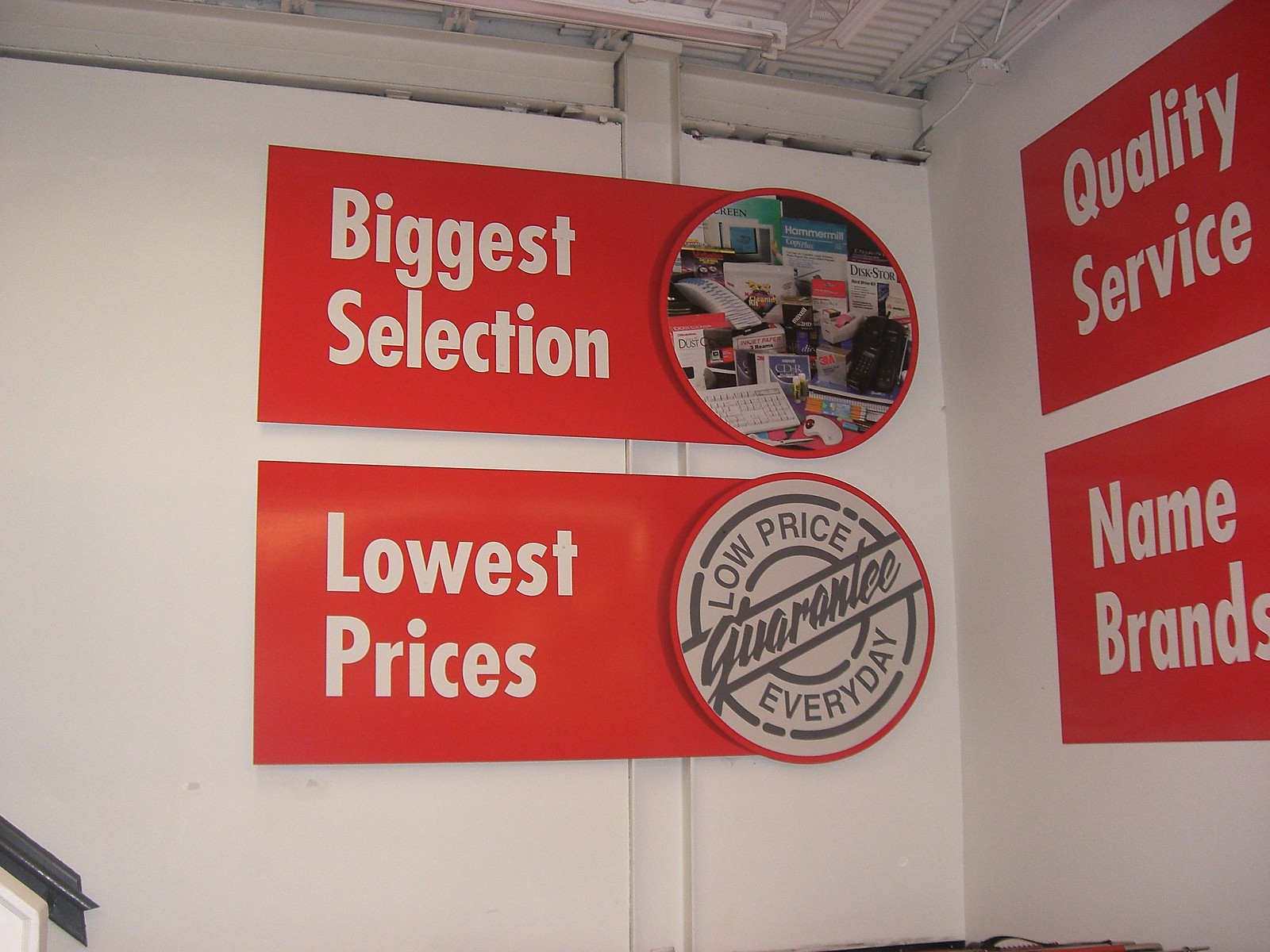This photograph captures the interior wall of an electronics store, featuring four prominent red signs with white lettering on a bright white wall, positioned in the corner of the room. The ceiling is constructed of corrugated metal and illuminated by hanging fluorescent strip lights. On the left facet of the wall, two rectangular signs are visible: the top sign reads "Biggest Selection," accompanied by a circular image displaying a variety of electronics, including keyboards, radios, telephones, and game controllers, all arranged on tables or boxes. Below it is the "Lowest Prices" sign, with a circular emblem stating "Low Price Guarantee Every Day." On the adjacent right wall, the top sign declares "Quality Service," with a second sign underneath proclaiming "Name Brands."